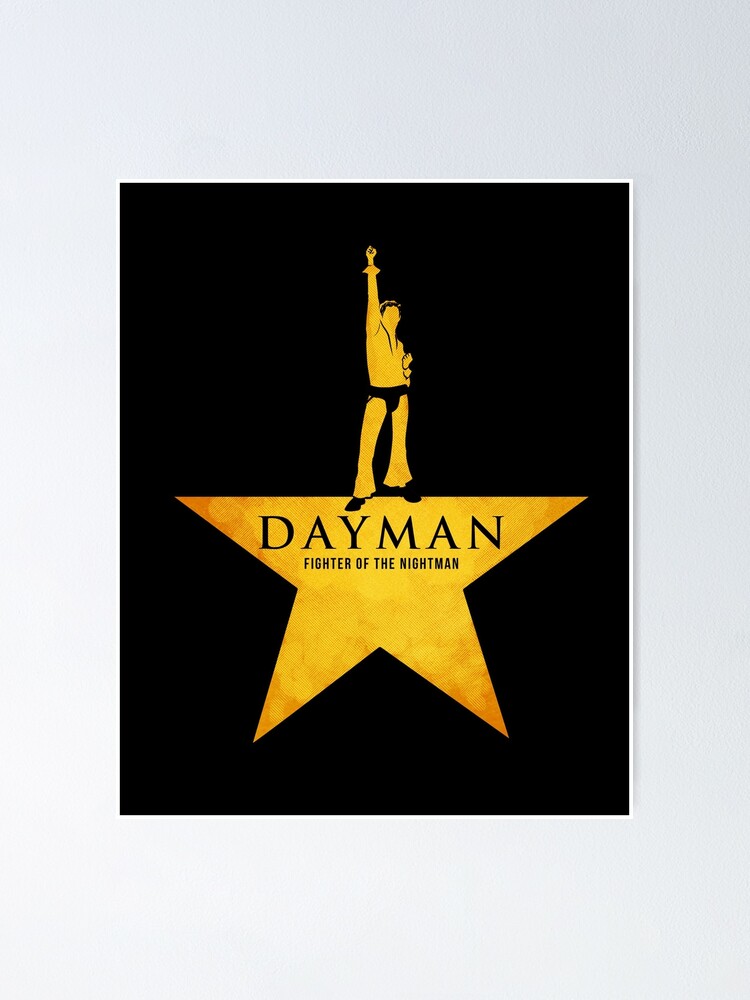A framed poster evokes the aesthetics of the Hollywood Walk of Fame, featuring a sleek black background with the bottom half of a glittering gold star at the center. Within the golden star, inscribed in bold black lettering, are the words "DAYMAN, Fighter of the Nightman." Above the star, a striking illustration of a man with black hair stands out. He is dressed in an outfit reminiscent of classic 70s icons, combining elements of both Elvis Presley and John Travolta's character from "Saturday Night Fever." The figure is posed dynamically, with his right hand dramatically lifted upwards. He sports bell-bottom pants, a black belt, and black shoes, capturing a sense of energetic performance or celebration. All of this is enclosed within a simple silver frame, making the entire piece a captivating blend of retro glamour and theatrical flair.